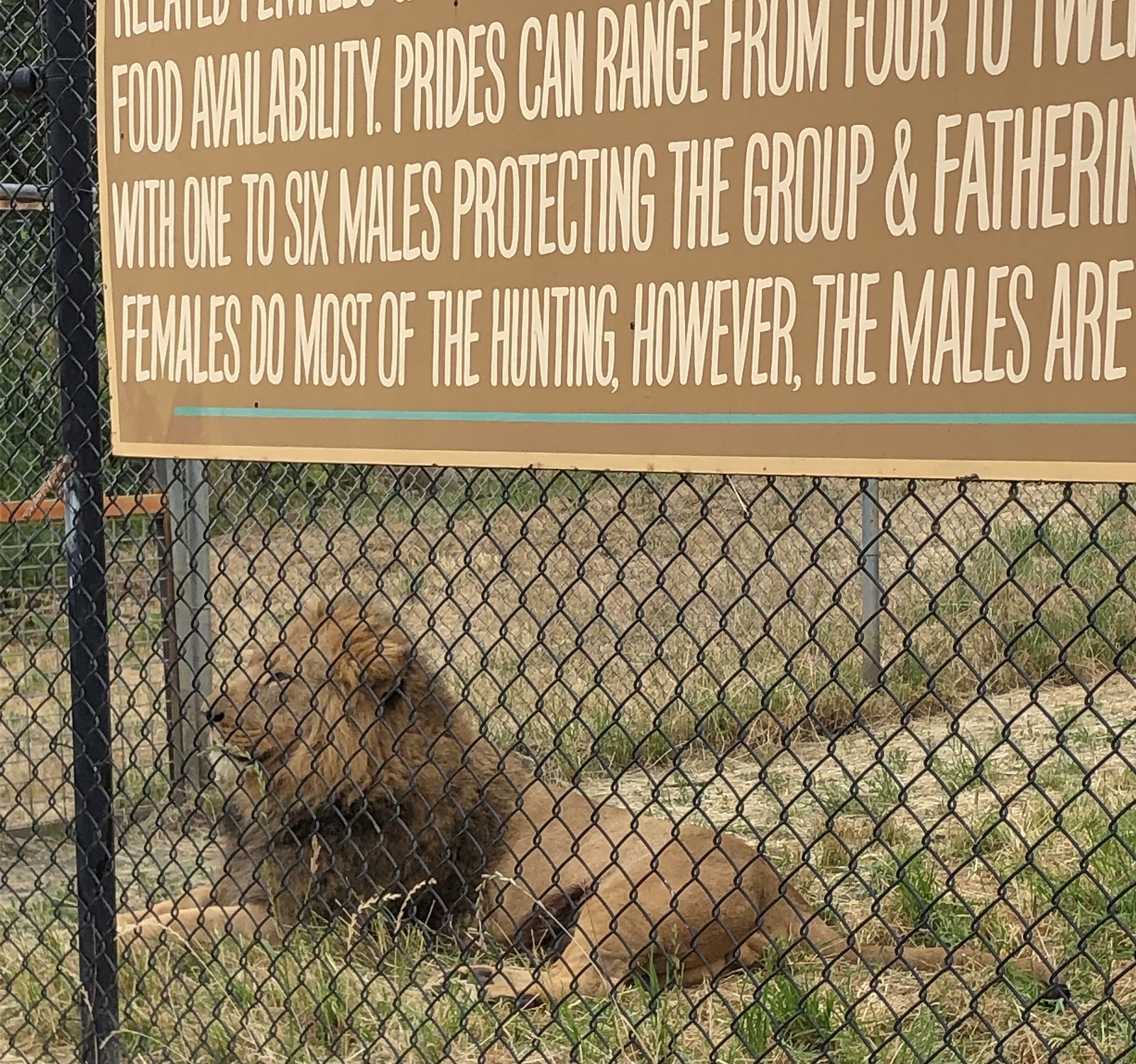This square-shaped photograph, likely taken at a sanctuary or zoo, captures a serene yet restrained scene featuring a majestic male lion lying down and gazing off to the left. Surrounding the lion is a chain-link fence, situated where two such fences converge, creating a corner enclosure. Above the lion is a partially visible large sign, predominantly brown with white text, that provides educational information about lion behavior and social structure. The legible portions of the text include phrases like "food availability," "prides can range from four to," and "one to six males protecting the group," alongside details about the roles of males and females within the pride. The background hints at a hot summer day, with mostly yellow, dry grass interspersed with sparse green patches, adding to the overall atmosphere of the enclosure.